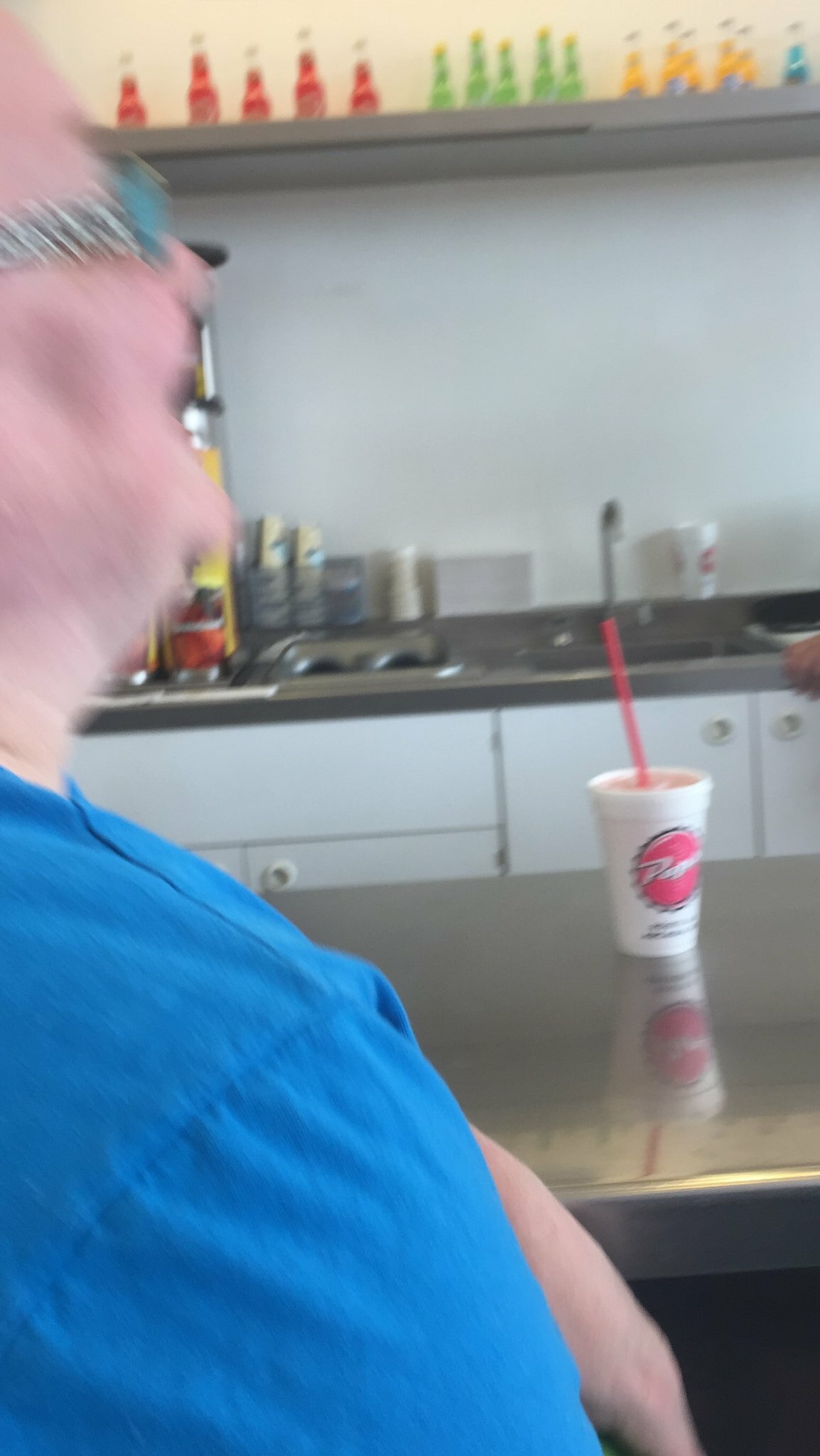In this slightly out-of-focus photograph, a bustling kitchen scene is captured. Prominently in the foreground, there is a hard metal table with a clear styrofoam cup placed on it, featuring a red straw and a red circular logo that appears to read "Peggy's" or another name starting with a 'P'. To the left of the cup, a person whose gender is indiscernible is seen in profile, their head blurred due to movement. They are wearing glasses and a blue shirt, and are turned slightly away from the camera.

In the background, a large sink is visible, accompanied by a sleek, gray metal shelf above it. This shelf is neatly stocked with various bottles, organized meticulously by color. There are five bottles each of red and green, and an additional six or seven bottles alternating between blue and yellow. This overall setup hints at a well-used and organized kitchen environment, possibly in a restaurant or cafe.